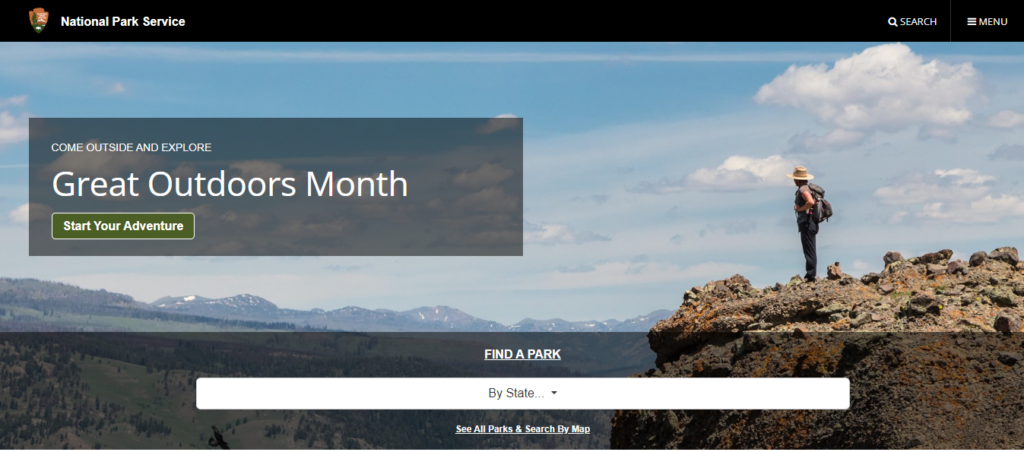The image showcases the National Park Service webpage, featuring a streamlined interface with a black bar at the top. On the left side, the National Park Service emblem is prominently displayed, alongside the text "National Park Service" in white. To the right, there is a search icon represented by a magnifying glass with the word "Search" next to it, followed by a menu icon in the form of three horizontal lines accompanied by the word "Menu".

Dominating the page is an inviting image of the great outdoors. The scene is a mountainous landscape, characterized by moderate elevations and a picturesque view. The mountain range is adorned with lush trees beneath a vibrant blue sky dotted with fluffy clouds. In the foreground, a solitary hiker with a backpack and a hat stands near the summit, gazing out at the breathtaking panorama.

On the left side of the image, a semi-transparent gray box overlays the sky, enhancing but not obscuring the scenic view. This box bears the inviting text, "Come outside and explore, Great Outdoors Month," followed by a button labeled "Start Your Adventure." Below it, another translucent gray box contains the phrase "Find a Park," which is hyperlinked for easy navigation. Beneath this is a white box centered with the text "By State," allowing users to access a list of national parks specific to their state. At the bottom, a prompt encourages users to "See All Parks and Search by Map," ensuring easy access to a comprehensive list of park locations.